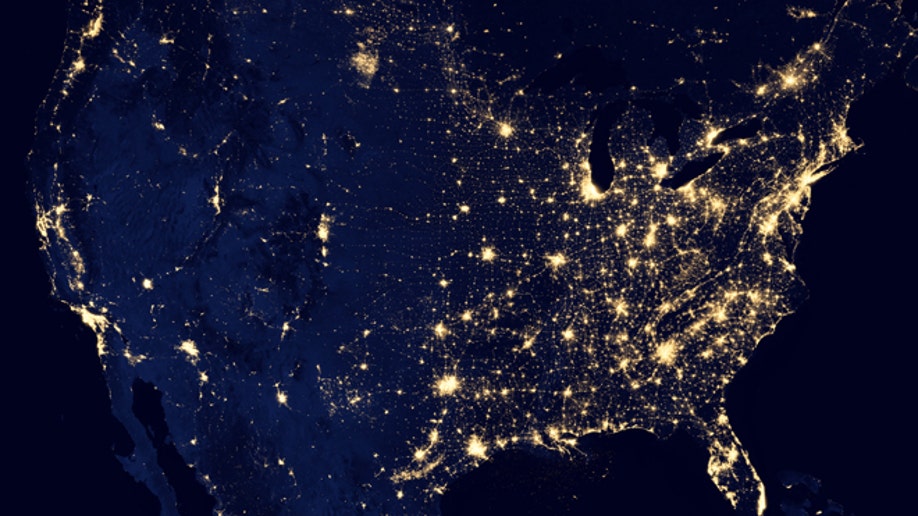This satellite image of the continental United States at night showcases the country illuminated by urban density and light pollution. Dominating the bluish-black background of the land, bright yellow lights cluster densely, particularly in major urban centers. On the East Coast, notable agglomerations of light mark New York City, Boston, Washington, D.C., Baltimore, and the surrounding areas, indicating higher population density. The Midwest features notable brightness around cities like Chicago and Michigan, with some spread of smaller, but still prominent, light concentrations.

As the image transitions westward, the light clusters become sparser, highlighting the vast, darker regions of rural America, especially evident in states like Utah and Nevada. Nonetheless, significant light patches are visible over western cities like Phoenix, Salt Lake City, and Denver. The West Coast similarly features considerable illumination over urban areas such as San Diego, San Francisco, and Los Angeles. Surrounding the landmass, the dark outline of water is distinctly black, providing a stark contrast to the illuminated continental landscape. The overall effect is a striking depiction of the United States' nighttime appearance from space, vividly illustrating areas of high and low urban density.